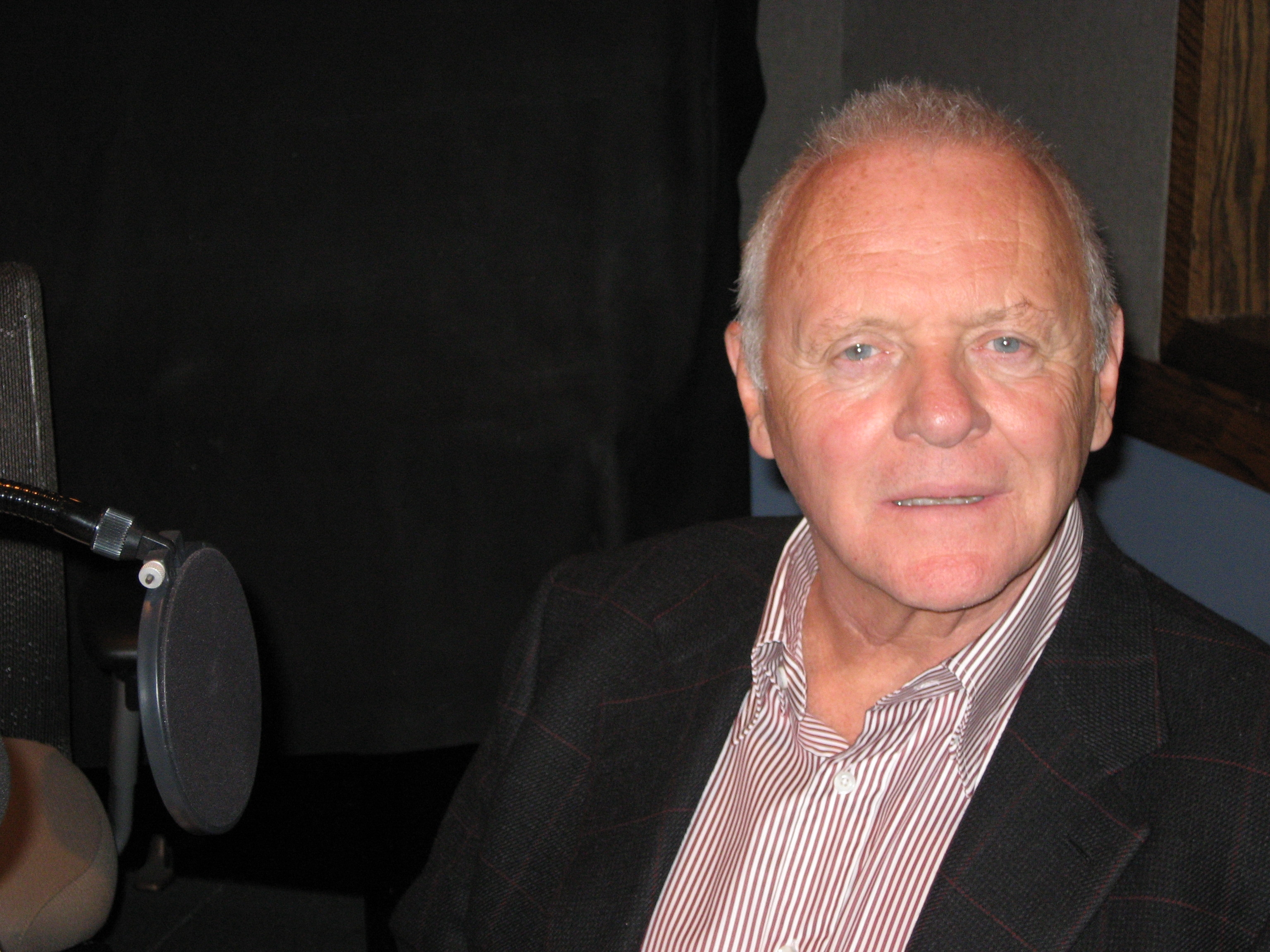In this image, we see the esteemed actor Anthony Hopkins, known for his role in "Silence of the Lambs." He appears slightly older, with short, stylish gray hair and striking blue eyes. He's clad in a black suit jacket over a strikingly pearlescent red and white striped shirt that’s buttoned up but open at the collar. Anthony Hopkins is seated in what seems to be a recording studio or radio station, characterized by a dark background and a gray wall, with a wood-grained window visible. A round, black microphone with a circular filter is prominently positioned in front of him, hinting that he might be recording or speaking. He gazes directly into the camera, slightly raising one eyebrow, and has his mouth partially open, as if he's about to speak. The ambiance is completed by the suggestion of a painting or portrait behind him, adding a touch of sophistication to the setting.